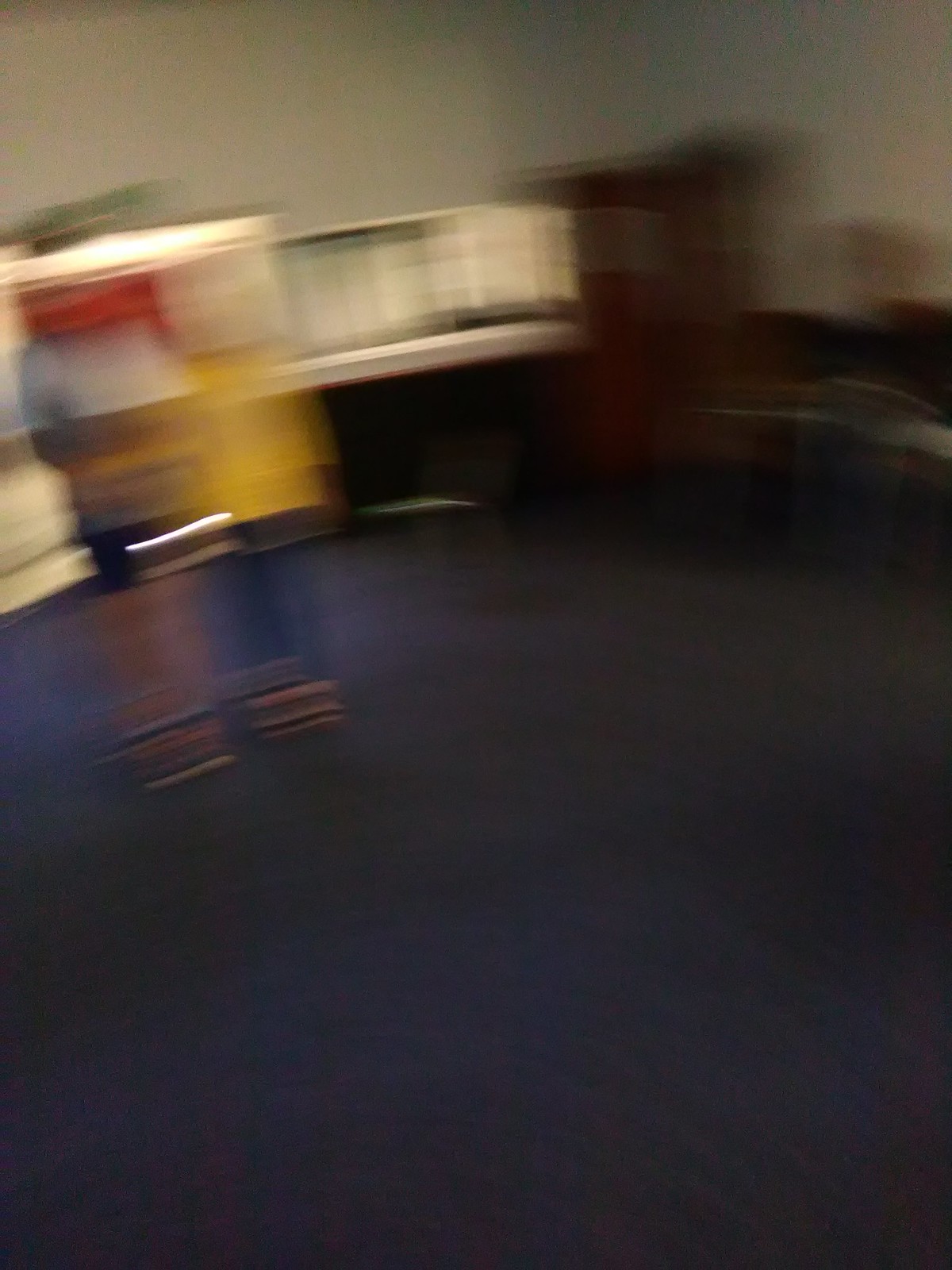A blurred vertical photograph captures an indoor scene, likely within an office setting. The space is characterized by blue carpeting and a large piece of brown furniture, possibly a computer desk, contributing to the office-like atmosphere. Despite the substantial blur and movement in the image, which obscure clear details, the center of the shot distinctly features an arrangement of square shapes in vibrant red, white, yellow, and blue hues. The dynamic, unfocused quality of the photograph lends an abstract, almost chaotic feel to the depiction of the office environment.